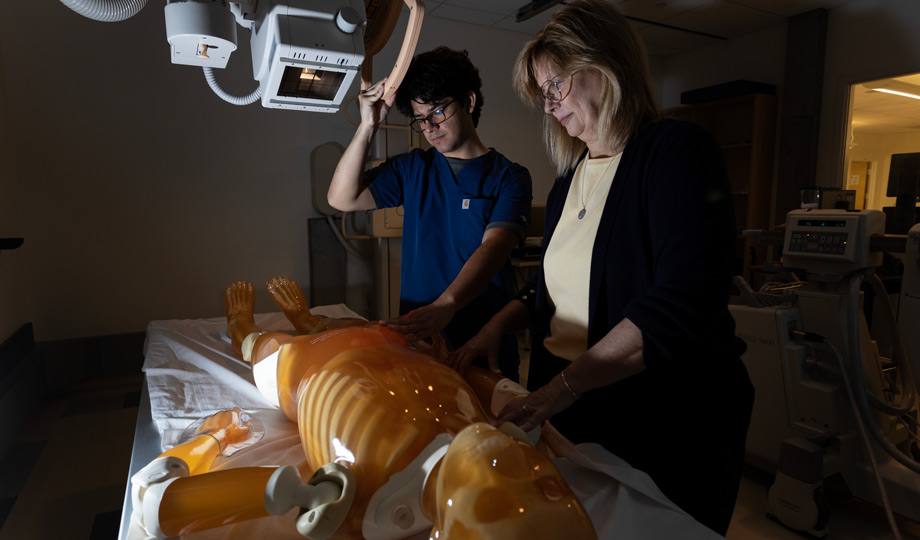The image is a horizontally aligned rectangular photograph capturing a medical room with various equipment and dim lighting, particularly on the right side. A strategically positioned window on the darker right side leads to another area. Centrally positioned is a hospital bed, angled diagonally, with a life-sized dummy resembling a human skeleton. The dummy has an orange and gold-colored coating, evoking the appearance of honey, highlighting its robotic features with visible bones on the head.

The background reveals medical equipment, with a white wall partially obscured by shadows. Above the bed, an x-ray machine is suspended from the ceiling, which a young man with short curly black hair and glasses is operating. He is dressed in a blue t-shirt, coordinating with his blue scrubs, and is captured in motion, adjusting the equipment. Beside him stands a woman with shoulder-length blonde hair, adorned with glasses and a slight smile. Her attire includes a black long-sleeved jacket over a yellow shirt and black pants, accessorized with a necklace.

Together, the man and woman intently examine the dummy on the hospital bed covered by a white sheet. In the background, additional medical apparatus enhances the clinical setting, reinforcing the scene as a modern medical or hospital environment.